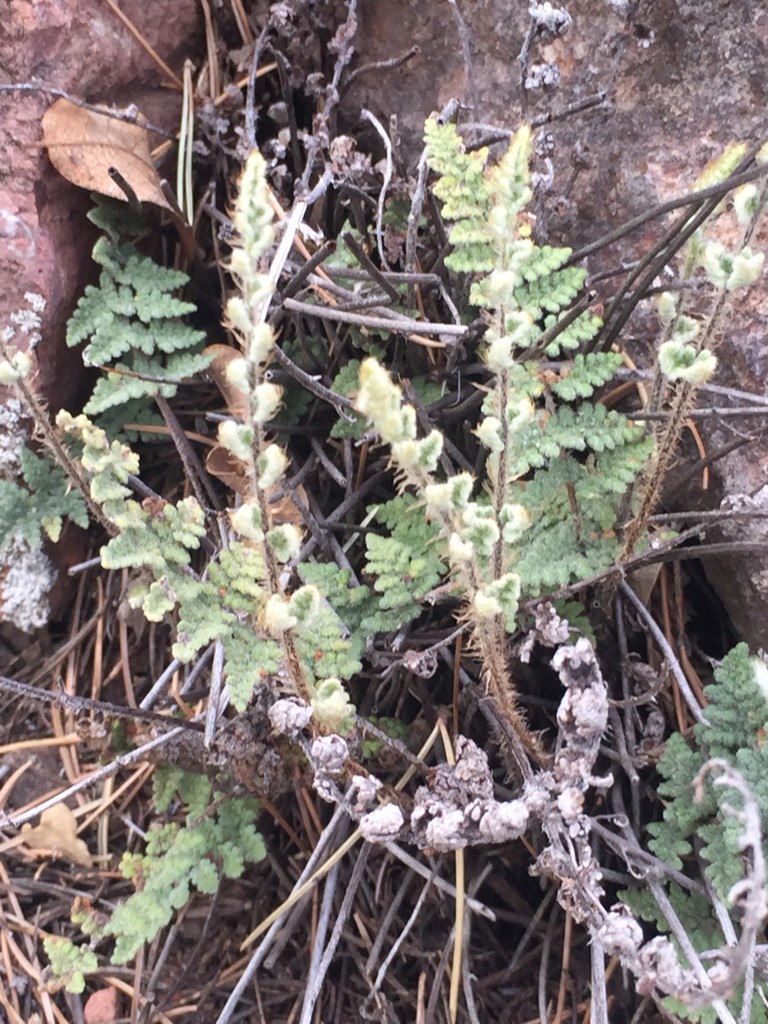This detailed and richly textured image captures the raw essence of untamed nature. Set against a reddish-brown, leaf-littered ground, a lush fern takes center stage, its greenery contrasting sharply with the earthy backdrop. The fern's multiple branches spread out, showcasing vibrant green leaves. Scattered beneath, dried sticks and stems form a tangled underlayer, adding to the image's complexity. In the lower right corner, a cluster of dried branches, adorned with white protrusions, adds a striking element of detail. The chaotic tangle of vines and sticks gives a sense of wild abandonment, while the faint presence of rock-like structures at the top corners grounds the scene in a more solid context. This photograph, likely captured spontaneously during a walk in the wild, encapsulates the rustic, unkempt beauty of nature—teeming with a medley of greens, whites, and browns, and brimming with a raw, organic charm.